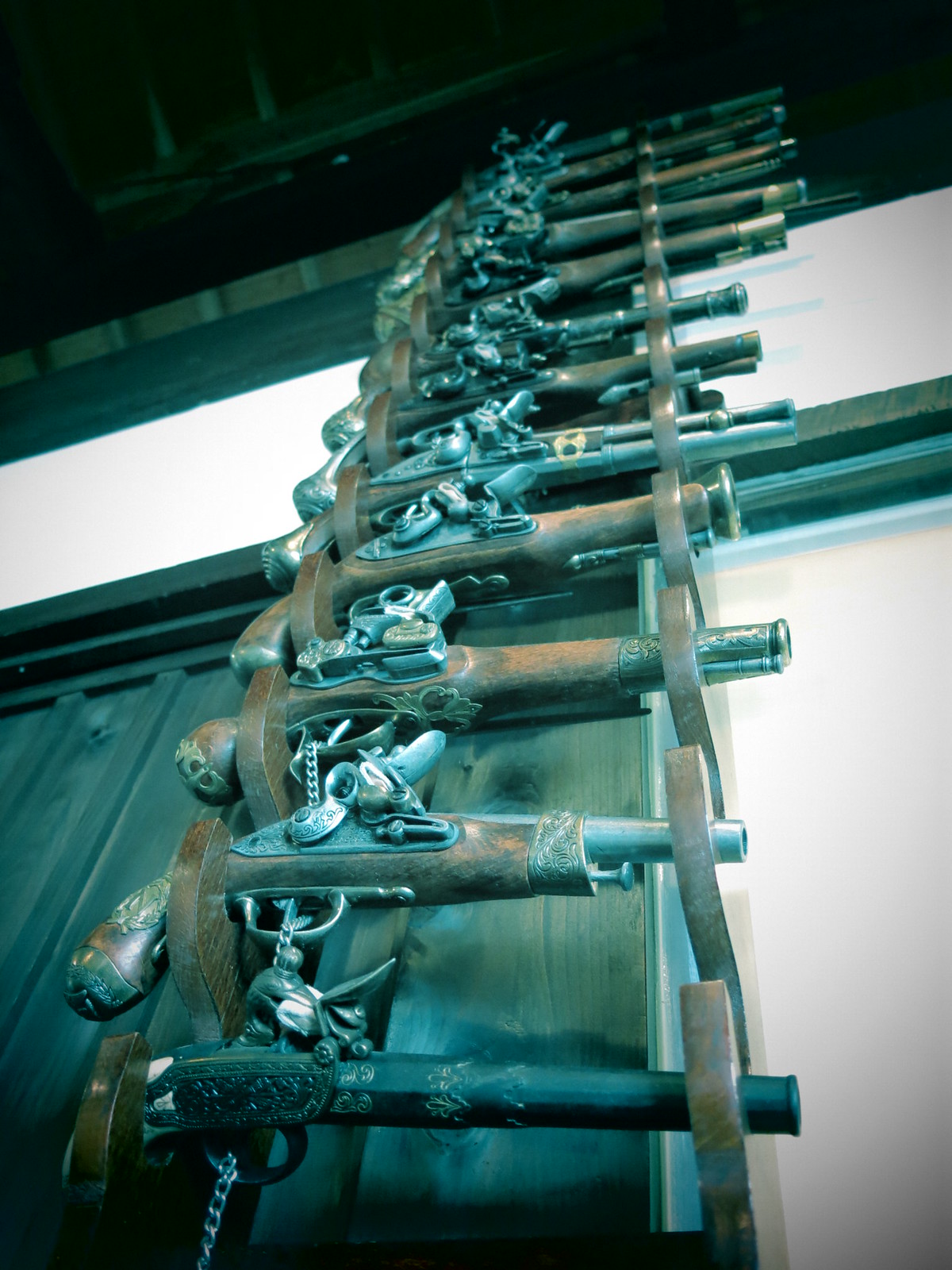The image showcases an extensive collection of flintlock guns displayed vertically from floor to ceiling on a brown wooden gun rack. These black powder firearms, resembling those carried by pirates in movies, exhibit a variety of designs and styles from different eras. Each gun features a long barrel, with many adorned with engraved metal work. Most of the guns have wooden handles shaped like small doorknobs, with metal caps at the end for loading powder. The collection is secured by a chain running through the triggers, and some barrels are covered for safety. The rack stands against a wall with dark-colored, possibly black or dark brown, ceiling and black trims, complemented by wooden trim in the middle. The collection is substantial, likely comprising over ten flintlock guns, each unique and rich in detail.